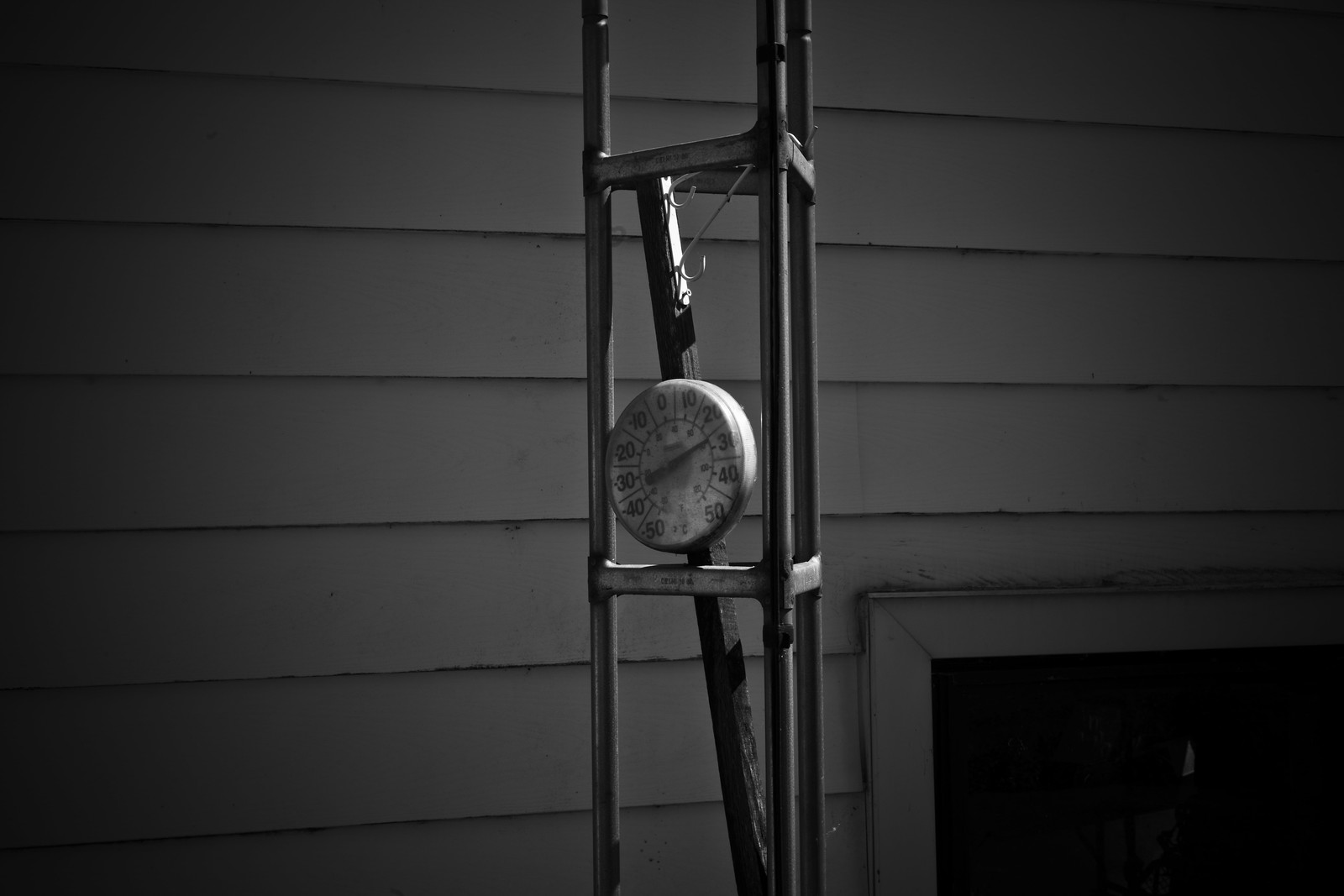This black-and-white photograph has a vintage feel, accentuated by a vignette effect that darkens the outer edges. Central to the image, a triangle of slender steel bars forms an intricate support structure. These bars, reminiscent of the size and delicacy of bird feeder stands, hold an outdoor thermometer. The thermometer, which features clock-like arms to indicate temperature, is housed within this steel frame. This frame is adorned with a decorative steel scroll in its middle section, adding an ornate touch. The triangle is divided into three sections by horizontal bars, further enhancing its architectural intricacy. In the background, the siding of a house is visible, with the bottom right corner of the photo featuring what looks like a cut-out frame, possibly for a window or door. The thermometer's needle points to a chilly 25 degrees, encapsulating the stark, cold ambiance of the scene.